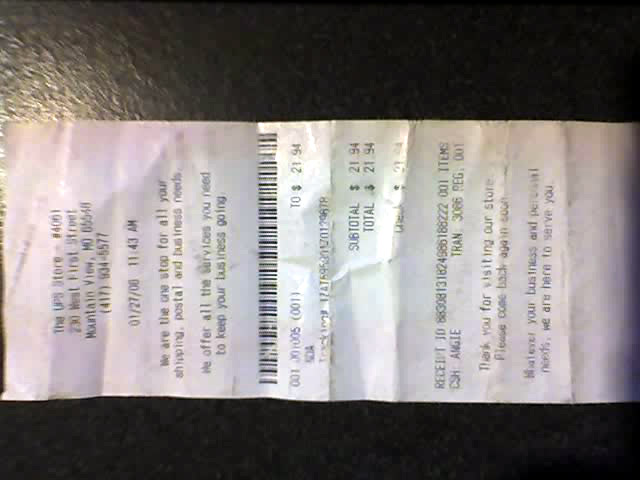The image displays a white paper receipt from the UPS Store #64001, located on West 1st Street in Mountain View, Missouri, ZIP code and phone number included. The receipt, dated January 27, 2006 at 11:43 AM, is for a package shipment costing $21.94. It appears in a horizontal layout against a black background, likely a kitchen counter or office desk, and has been folded in an accordion style, leaving prominent vertical creases. The receipt contains black text and a barcode situated about two-thirds down its length, turned perpendicularly so that its top faces the left side of the image. Despite the intricate folds, the entire length of the receipt is visible with no other objects or text present in the photo.